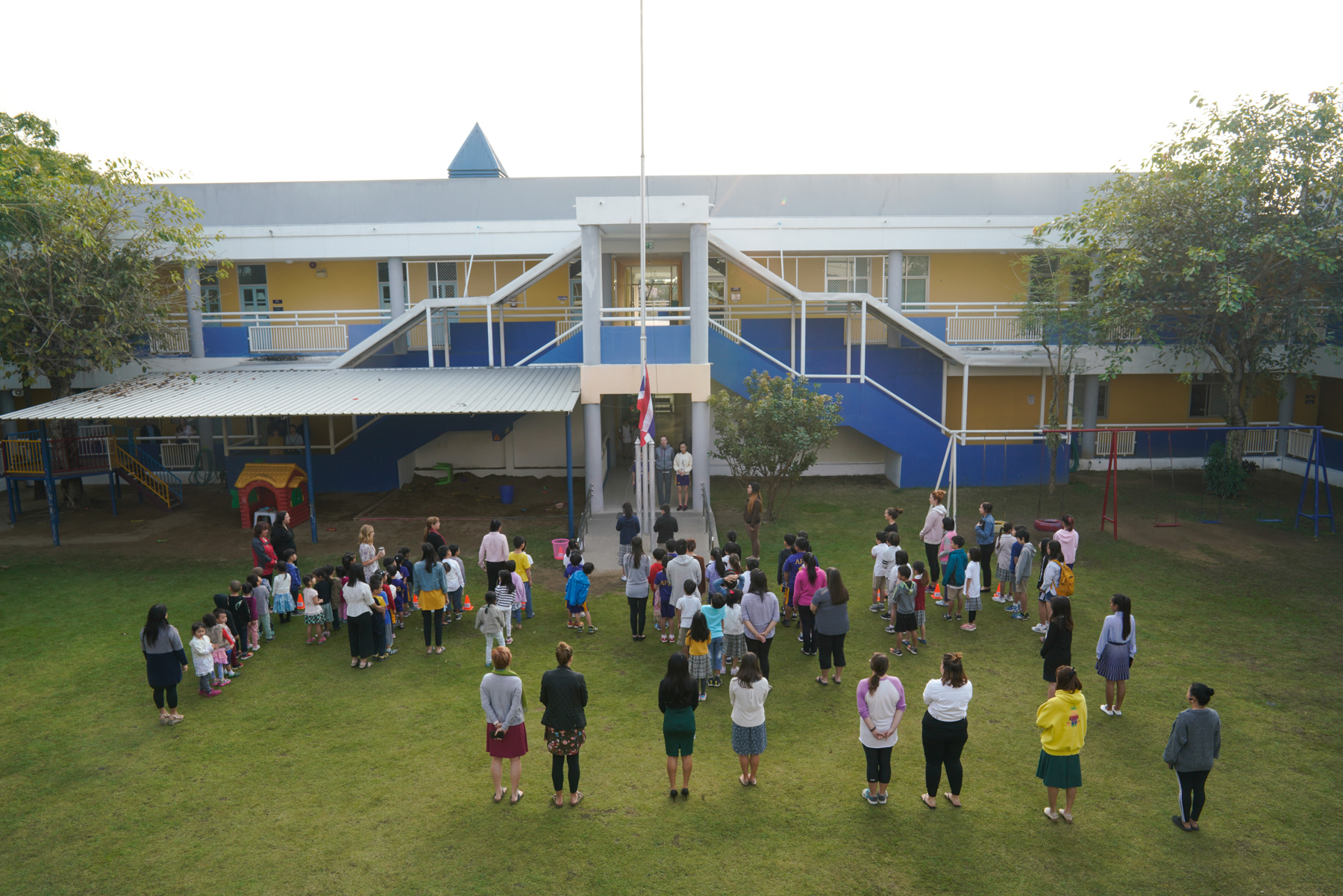This photograph captures a flag hoisting ceremony at an elementary school. The scene is set in the school's courtyard, adorned with a building painted in yellow with blue trim and featuring a blue stairwell on the left side. In the center of the image stands a flagpole, with a partially visible flag in red, white, and blue, which may not be the American flag, possibly resembling the Union Jack. The courtyard is surrounded by greenery, including well-manicured grass and several trees. To the right, there are sets of swing sets painted in red, white, and blue, and a small playground with equipment such as a tire swing and a small red house with green windows and a yellow roof. A large gathering of students and teachers, dressed in various colors, are assembled in rows on the grass, all facing the flagpole, possibly preparing for or engaging in a ceremonial activity like a Pledge of Allegiance.